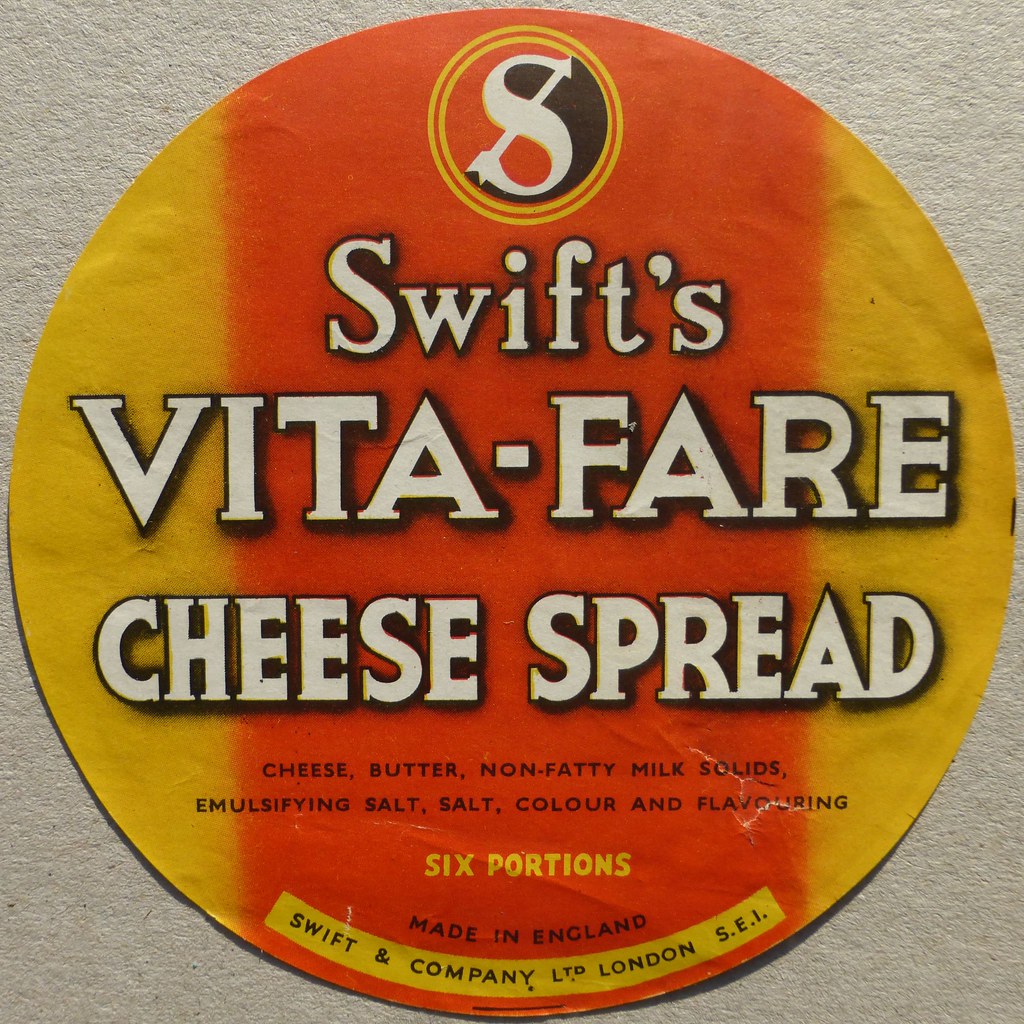This square-shaped image showcases a textured light beige background with a circular, slightly crinkled label as the main subject. The label's vibrant gradient shifts from a bright burnt orange in the center to yellow on the left and right edges. At the top of the label, a smaller yellow circle, encased in golden and red bands, features a stylized white letter "S" with an arrow through it, denoting the brand’s logo. Below the logo, in prominent white font with thick black shadows, the text reads "Swift's Vita Fair cheese spread" across three lines: "Swift's" on the first, "Vita Fair" on the second, and "cheese spread" on the third. The label further details the product in a smaller, yellow font, listing ingredients such as "cheese, butter, non-fatty milk solids, multiplying salt, salt, color, and flavoring". Additional text includes "six portions" and "Made in England" in dark font. At the bottom, in black letters on a tannish yellow background, it states "SWIFT AND COMPANY, LTD. London, S.E.I." The descriptive and sharply contrasting color scheme makes this cheese spread label both eye-catching and informative.